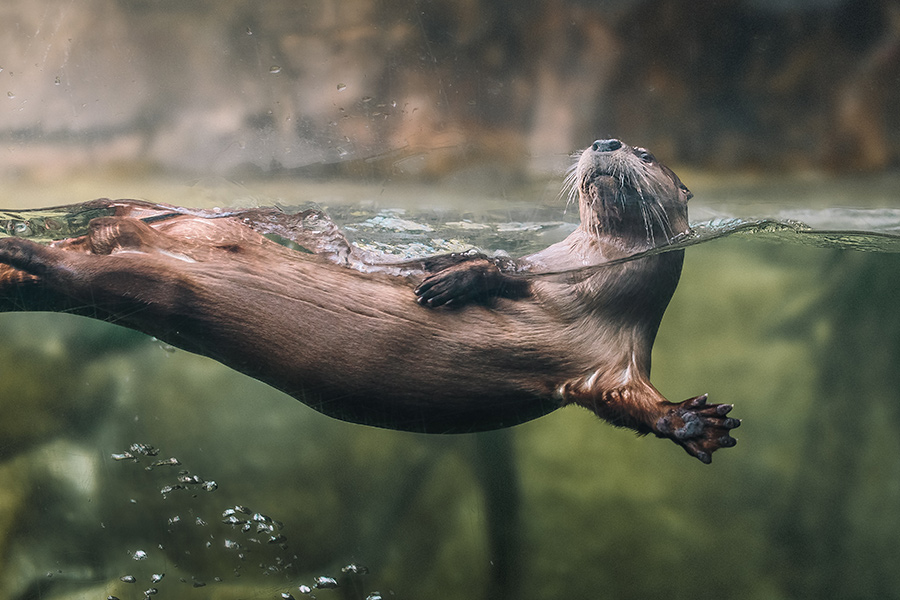This is a detailed horizontal rectangular photograph of a river otter, captured in mid-swim with a striking mix of underwater and above-water elements. Positioned mostly underwater, the otter's body is a rich brown, while its head and neck, which stick out of the water, have a grayer hue. The otter lies on its back and stretches one arm forward underwater, while the other is folded against its side. Its legs are visible along with its outstretched tail, and it gazes upward, head partly lifted. Notably, the otter's face is adorned with a profusion of long white whiskers, particularly noticeable around its nose. The water, a somewhat clear yet murky green, reveals bubbles and reflections from the shoreline above. These reflections hint at a leafy, tree-lined environment, enhancing the natural, verdant backdrop in the photograph. Blurry trees and plants both above and below water add depth and context, highlighting the otter's serene, almost playful presence.